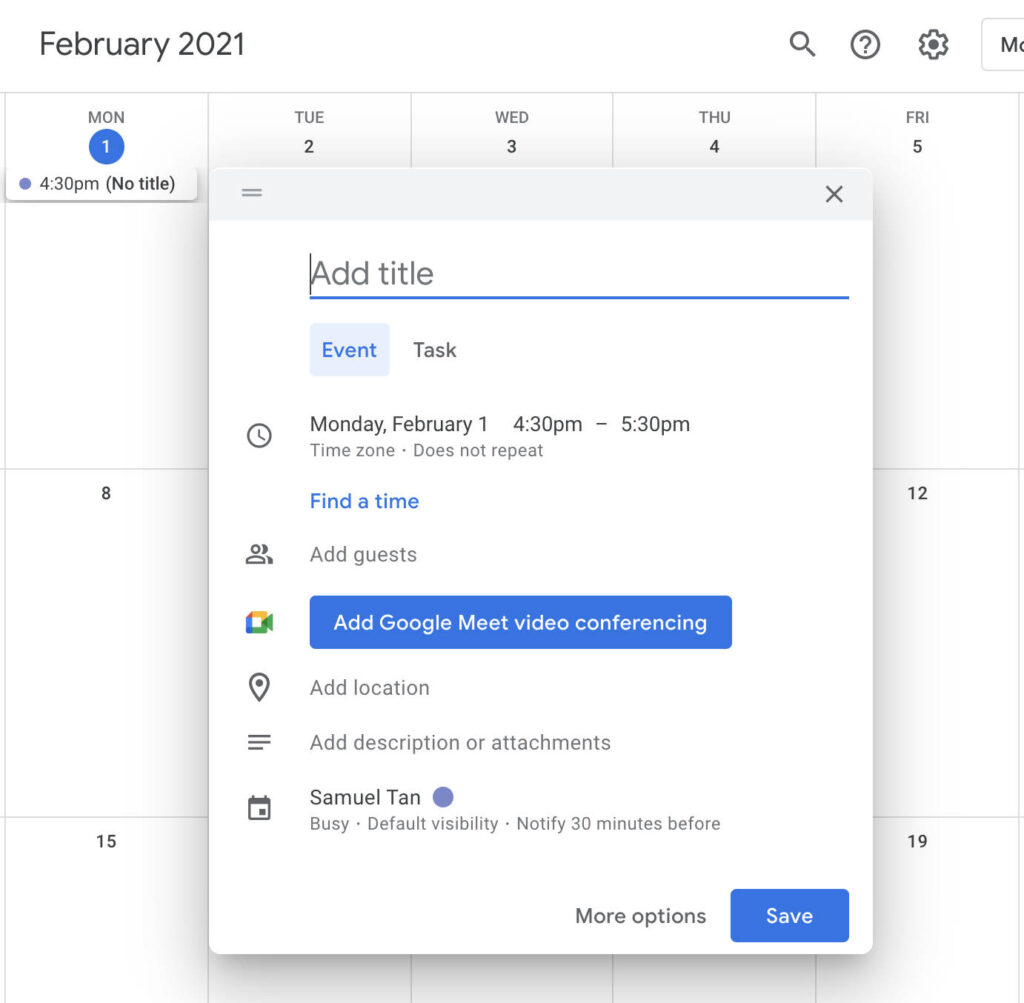A screenshot of a digital calendar for February 2021 is displayed, showcasing days of the week including Monday, Tuesday, Wednesday, Thursday, and Friday. Specific dates such as the 2nd, 3rd, 4th, 5th, 8th, 12th, 15th, and 19th are visible. A single date is highlighted in blue, indicating a scheduled event on Monday, February 1st, from 4:30 p.m. to 5:30 p.m. 

A pop-up screen is open that prompts the user to add an event. It lacks a title and offers options to add details such as event title, task, location, description, or attachments. There are also links to find a suitable time and add guests. The user can add Google Meet video conferencing for the event. The default visibility is set to 'Busy' and notifications are set to go out 30 minutes before the event. The username "Samuel Tan" is associated with the calendar entry.